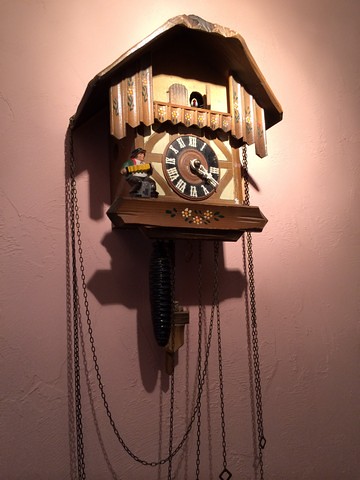The image features an old-fashioned, wooden cuckoo clock mounted on a pink painted wall illuminated by some light. The clock is designed to resemble a rustic house with a pointed roof. At the top, there is a small window with curtains and a door, half open, where the cuckoo bird emerges. Below this, at the lower level, is the clock's face, which is circular with an outer brown color and black background. The clock displays white Roman numerals and currently shows the time as 4:20. The hands of the clock are all pointing in one direction. On the left side of the clock, there's a wooden carving of a man playing an accordion. The clock mechanism is complemented by chains on its sides for setting and resetting the time.